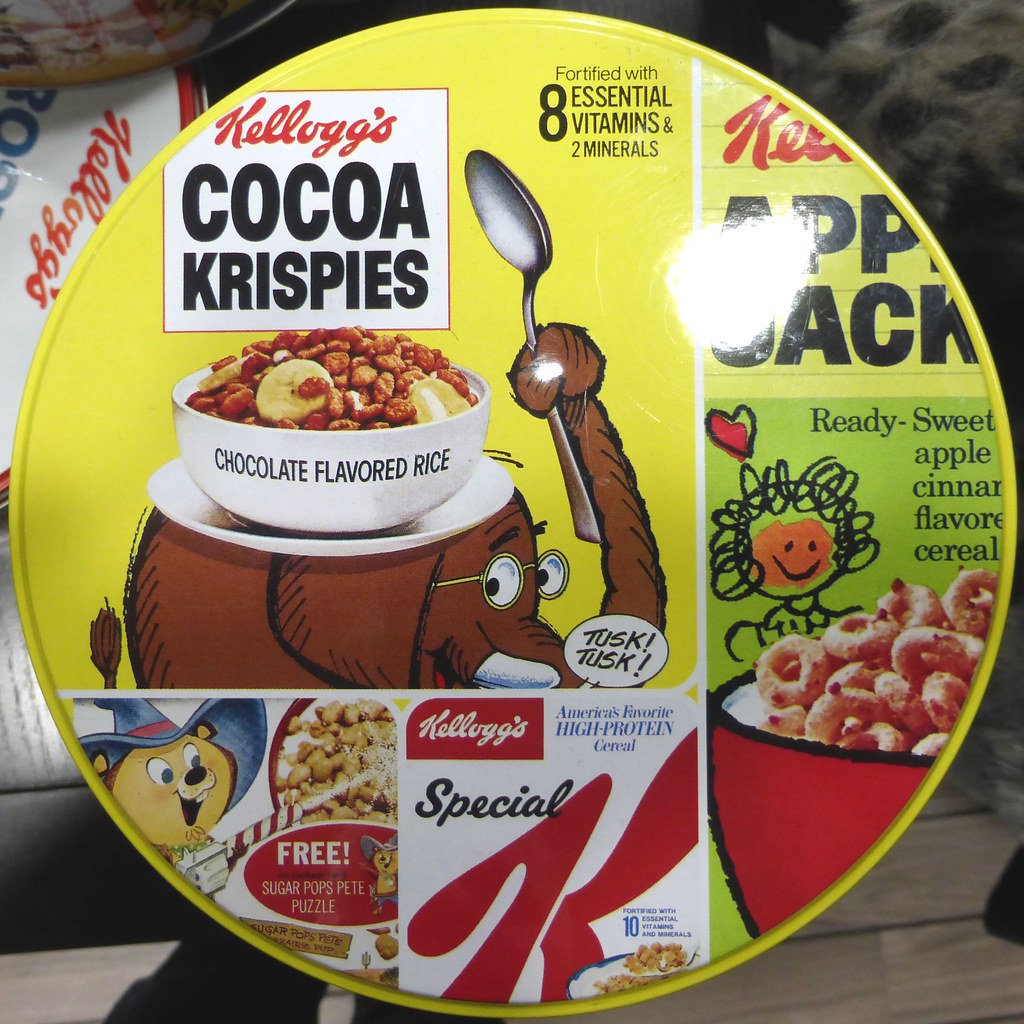This image features a top-view photograph of a circular cereal cup lid divided into distinct sections. Dominating the top-left section is the label for Kellogg's Cocoa Krispies, showcasing a cartoon brown elephant with glasses holding a spoon. The elephant is perched beside a white bowl filled with chocolate-flavored rice cereal. Adjacent to this, on the upper right segment, partially visible due to cropping, is the label for Kellogg's Apple Jacks. It includes a depiction of a stick-figure girl with curly hair staring at a red cereal bowl, accompanied by the phrase "Ready Sweet Apple Cinnamon Flavor." The bottom portion of the lid highlights Kellogg's Special K, proclaimed as "America's Favorite High Protein Cereal." This section also features a small character, possibly a mouse or bear, in a wizard hat gazing at a milk carton, with the text "Sugar Pops Pete Puzzle" nearby. A prominent banner on the upper right announces the inclusion of "8 Essential Vitamins and 2 Minerals." Overall, the vibrant, detailed design emphasizes the diversity of Kellogg's cereal offerings.